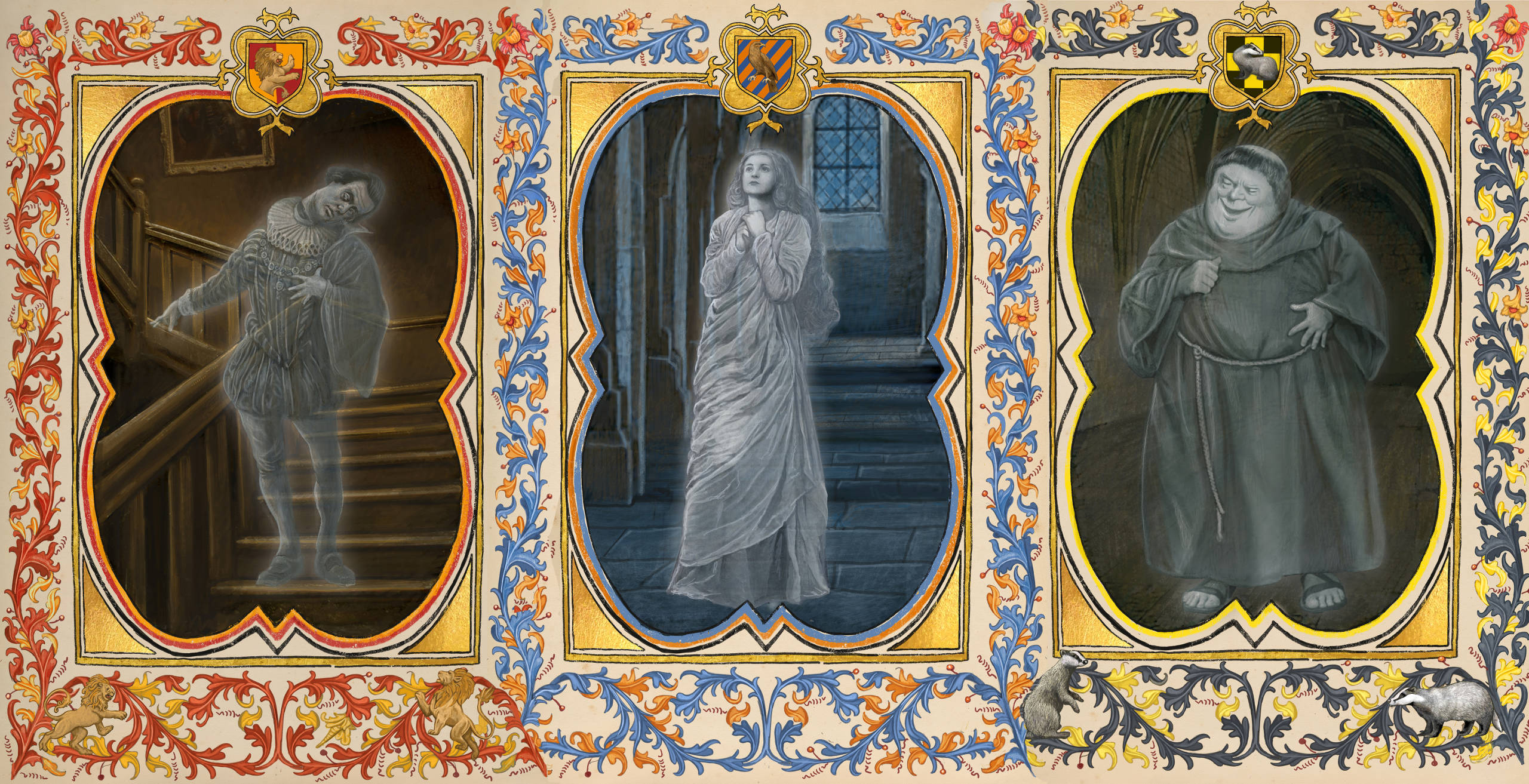A rectangular poster, divided into three distinct sections, captures your attention with its intricate design. Each section resembles a mini poster with a unified thematic representation. 

The background of the poster is a soft beige, providing a neutral canvas for the vibrant artwork within each segment. The right section is adorned with elaborate gold and red swirls and leaves, conjuring images reminiscent of Gryffindor from Harry Potter's Hogwarts houses, with a ghostly figure whose head appears slightly detached, evoking the spectral essence of Nearly Headless Nick.

The middle section stands out with its blue background, featuring a ghostly bird-like figure that exudes an ethereal demeanor. This spectral character, with hands gently clasped in front, hints at wisdom and tranquility, possibly drawing a parallel to the Ravenclaw house.

The left section contrasts the others with its striking black and yellow hues. Dominating this area is a jovial, rotund ghost, captured in a moment of hearty laughter. This spirited character might be an artistic representation intended to evoke the cheerfulness associated with Hufflepuff, completing the trio of houses.

Overall, the poster intricately blends colors and ghostly imagery to evoke the essence of the Harry Potter series, with each section thoughtfully designed to hint at the characteristics of different Hogwarts houses.